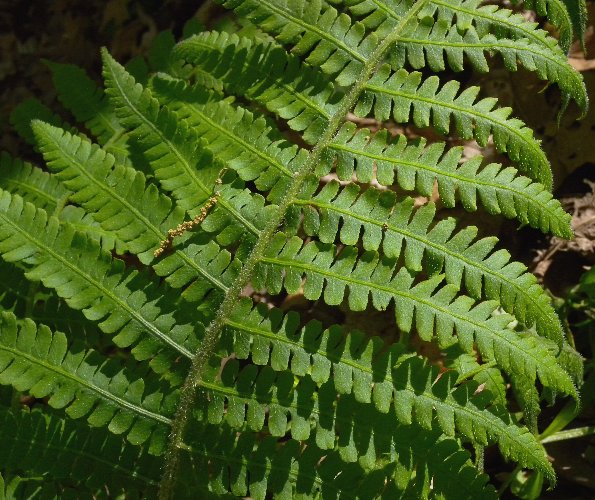This extreme close-up photograph captures the intricate details of a large, lush, dark green fern-like leaf. The central stem of the leaf, thick and prominent, extends vertically through the middle. Each branch of the leaf is lined with numerous spiky leaflets, which cast shadows onto the other parts of the leaf, highlighting its textured surface. Tiny droplets, possibly dew or moisture, cling to the leaflets, suggesting either a recent rainfall or a humid environment. On the leaf rests a few small particles, perhaps seeds or some other material. The backdrop consists of an indistinct brownish material, likely other leaves or organic matter, emphasizing the rich green of the primary leaf. The entire composition is strikingly detailed, emphasizing the natural beauty and complexity of the foliage.